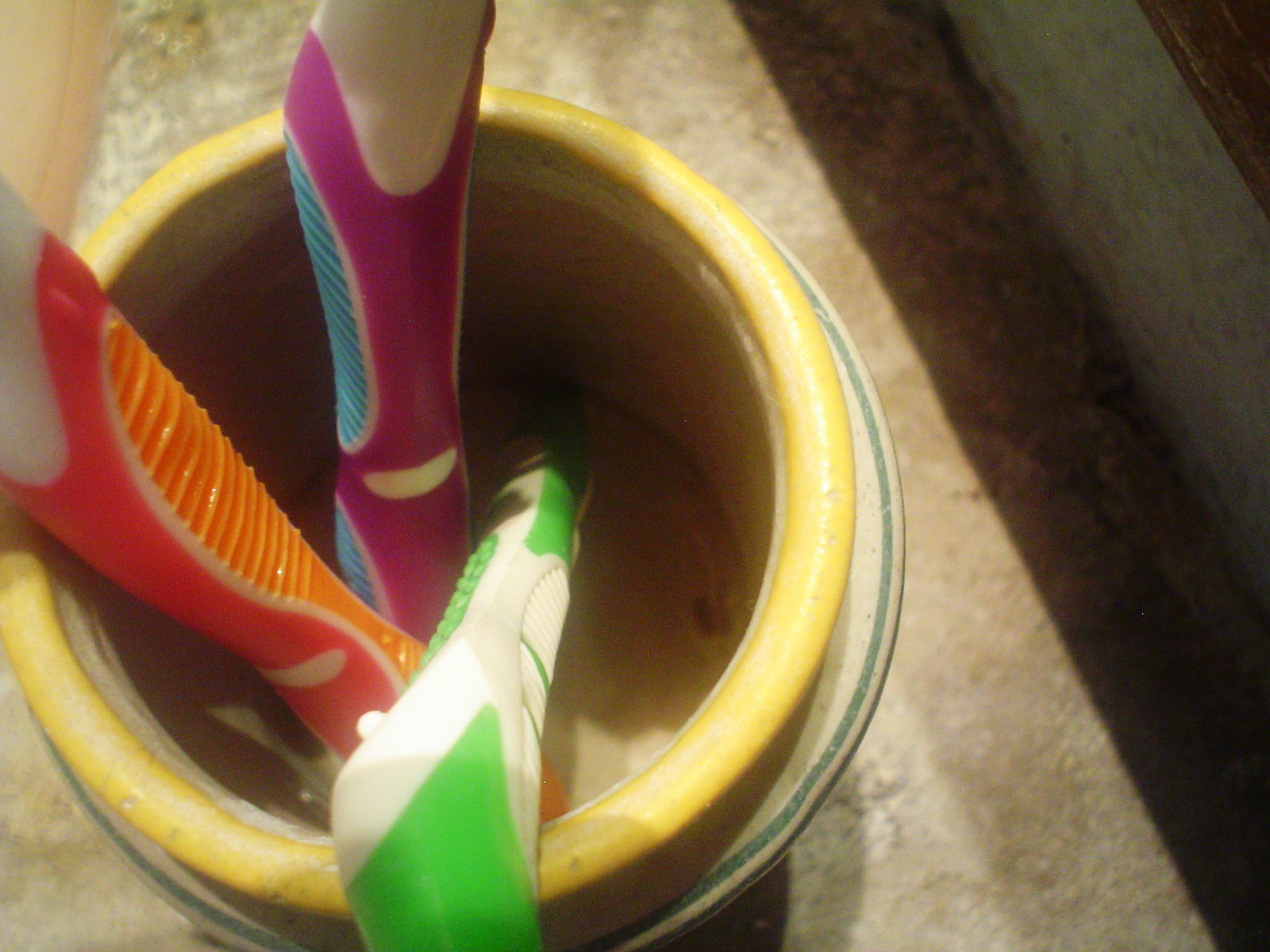This close-up photograph features a yellow cup with a beige interior, placed on a reflective brown marble countertop. The cup holds three toothbrushes, each boasting distinct colors and designs. The first toothbrush has a purple and white spotted body with a blue grip area. The second toothbrush displays a lime green grip with a white handle. The third toothbrush, positioned close to the others, features an orange grip with red accents, a pinkish-red body in the light, and a small white line between the grip and the brush head. The countertop casts a prominent shadow to the right, tapering nearer to the cup. This scene is a vivid display of daily essentials against a sleek, reflective surface.